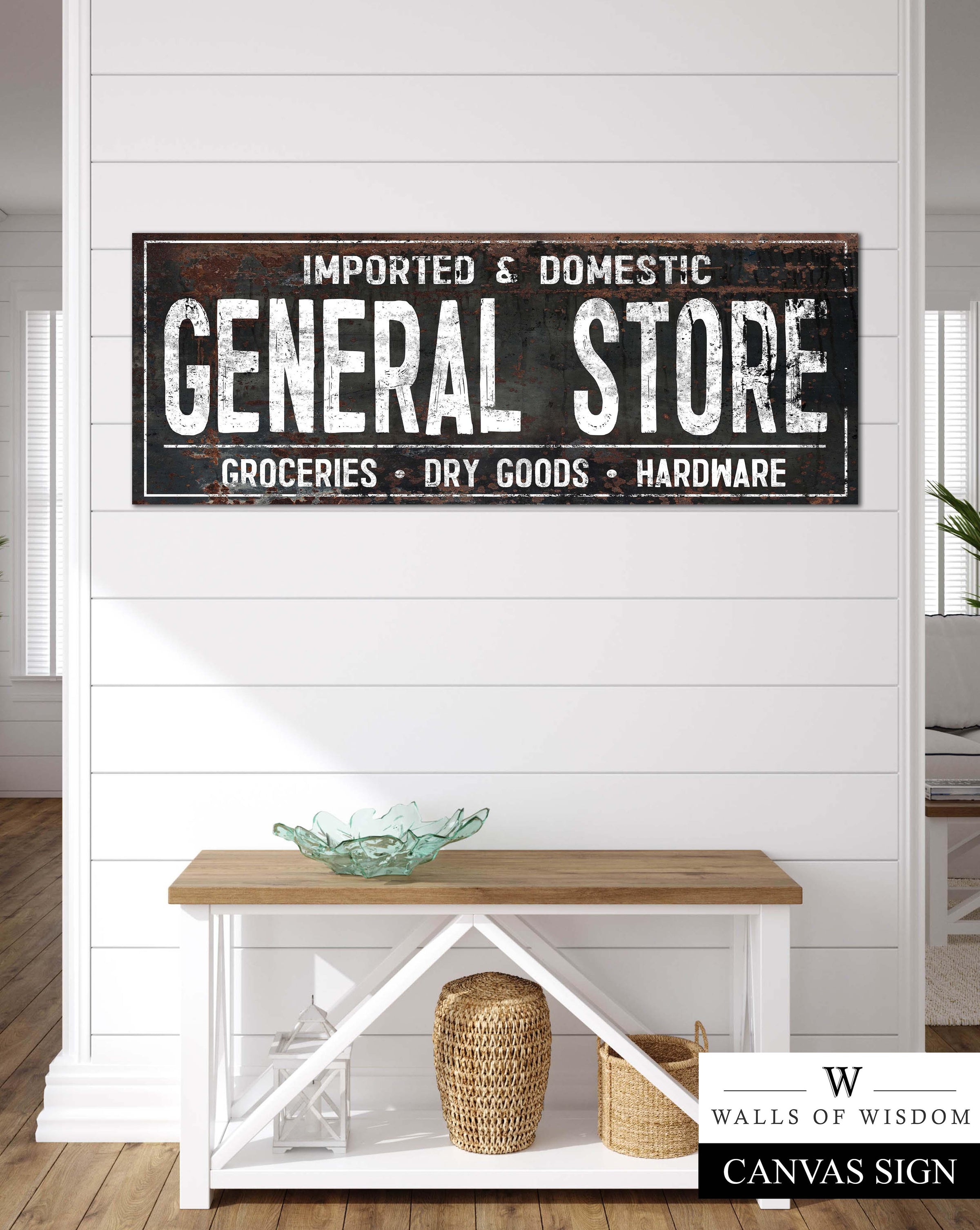The image showcases a vintage-themed room, possibly a living room or foyer, dominated by a large white-paneled wall that hosts an old, weathered sign. The sign, positioned above center, prominently displays in large white letters "Imported and Domestic" at the top, followed by "General Store" beneath it, and a white line separates this from the smaller text below listing "Groceries, Dry Goods, Hardware." This sign spans the width of the wall, adding a rustic charm to the room. Below the sign, there is a small table with a wooden top, white structure, and a base shelf. The table is adorned with decorative items including a glass bowl, a tissue box, a small wicker basket, and another small basket. The setting is warmly lit, featuring brown wooden flooring and windows that can be observed to the left and behind the wall. The bottom right corner of the image includes a partial view of a "Walls of Wisdom" canvas sign with a black "W" logo, adding to the room's vintage charm.